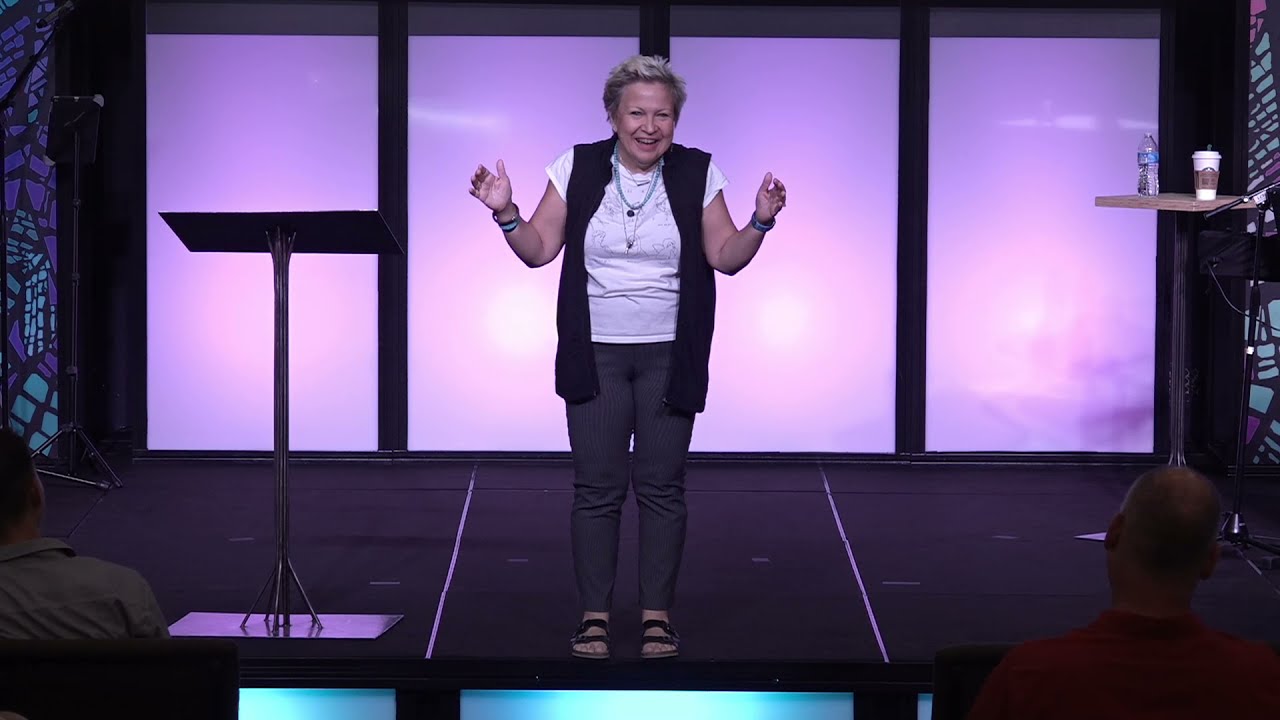The image captures a middle-aged woman on a black stage, seemingly in the midst of addressing a crowd, possibly telling a story or a joke. She is wearing a black sleeveless vest over a white shirt, paired with dark gray pants and black sandals. Her short blonde hair is neatly cropped, and she has wristbands on both wrists. Behind her, there are large, purple-lit door-sized windows or panels creating a striking backdrop. On stage to her left is a metal stand resembling a podium, possibly holding notes. Further back on the right side of the stage, there is a wooden table with a bottle of water and a white coffee cup. The audience includes a man with no hair wearing a red shirt and another person in a gray shirt with dark hair. The stage is further accentuated by blue and purple lighting elements on the front and far left side.